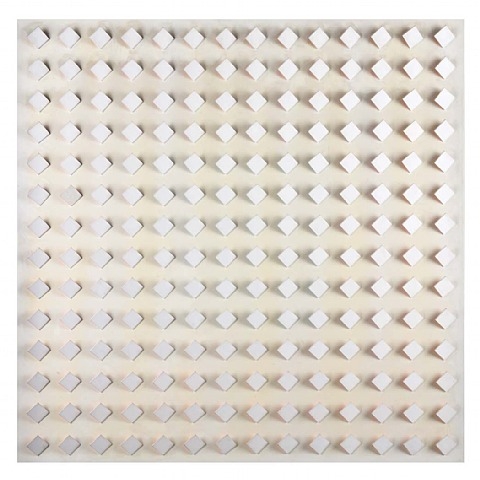This image is an abstract photo that resembles a painting, depicting an art piece with a meticulously arranged grid of diamond shapes. The background is a white board, onto which 14 columns and 14 rows of identical diamond shapes are mounted. Each diamond, appearing possibly as paper or small wooden pegs with a uniform square form turned on its side, creates a dynamic pattern across the white surface. The light source, seemingly from one side, casts delicate shadows behind each diamond, adding depth and dimension to the piece. The center of the art piece has a yellowish hue, transitioning to grayish tones towards the edges and corners, enhancing the overall texture and visual interest.